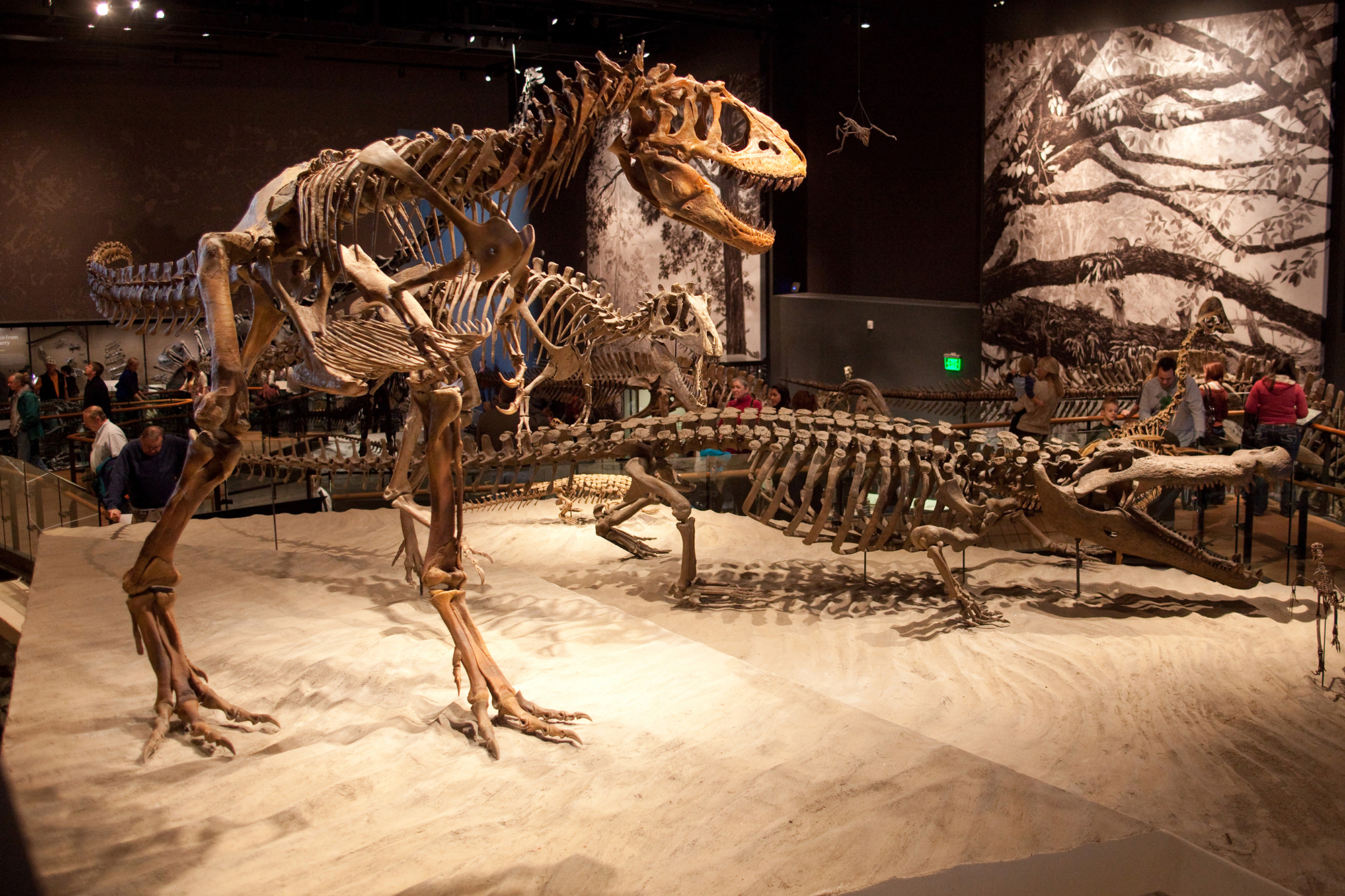In this museum exhibit photograph, we see two impressive dinosaur skeletons displayed on a sandy ground. To the left, the towering skeleton of a T-Rex stands upright on two legs, its small arms positioned in front and its mouth wide open, displaying an imposing presence. The bones exhibit a light brown to yellow color, capturing the attention immediately. On the right, a long skeleton resembling a crocodile or alligator stretches out on all four legs, characterized by an elongated body, a long tail, and a large, crocodile-like mouth, with similarly colored bones. The exhibit is surrounded by a guardrail, blending into the dimly-lit area, with people visible in the background on all sides. Above, from the ceiling, several small white lights shine down, emphasizing the skeletons amidst the dark backdrop. Further contributing to the scene, a large, black-and-white painting of tree branches and leaves hangs in the background, and to the right, a green illuminated box can be spotted above the alligator-like skeleton. Overall, the room maintains a subdued ambiance, directing focus onto the detailed and fascinating dinosaur skeletons.